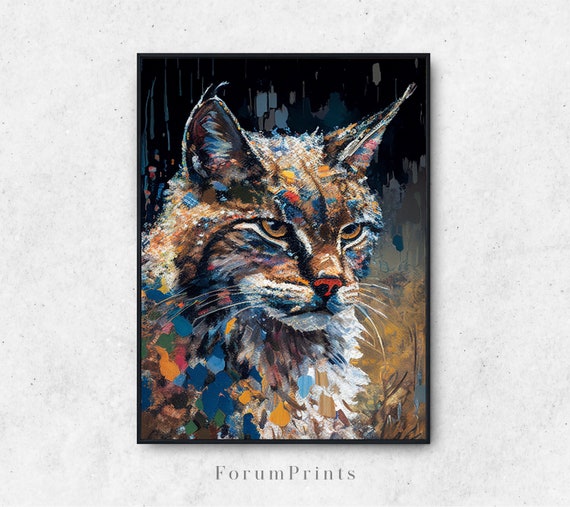This image features an expressive oil painting of a lynx cat, prominently displaying its head, throat, and upper chest against a predominantly black background with varying splashes of color. The lynx, facing towards the right, has striking yellow eyes and a pink nose. Its fur showcases a multitude of colors, including yellow, blue, pink, green, brown, beige, and white, giving it a vibrant and dynamic appearance as if paint were skilfully splattered all over. The lynx’s ears have characteristic tufts, adding to its wild charm. The artist meticulously painted white whiskers, with around four to five on each side. The background of the piece transitions from black and gray hues at the top to a mix of brown and blue towards the bottom right. Highlighted text at the bottom states "FORUM PRINTS" in light gray letters, possibly indicating the name of the print series or the company. The overall composition creates a striking and richly colored portrayal of this majestic wild cat.